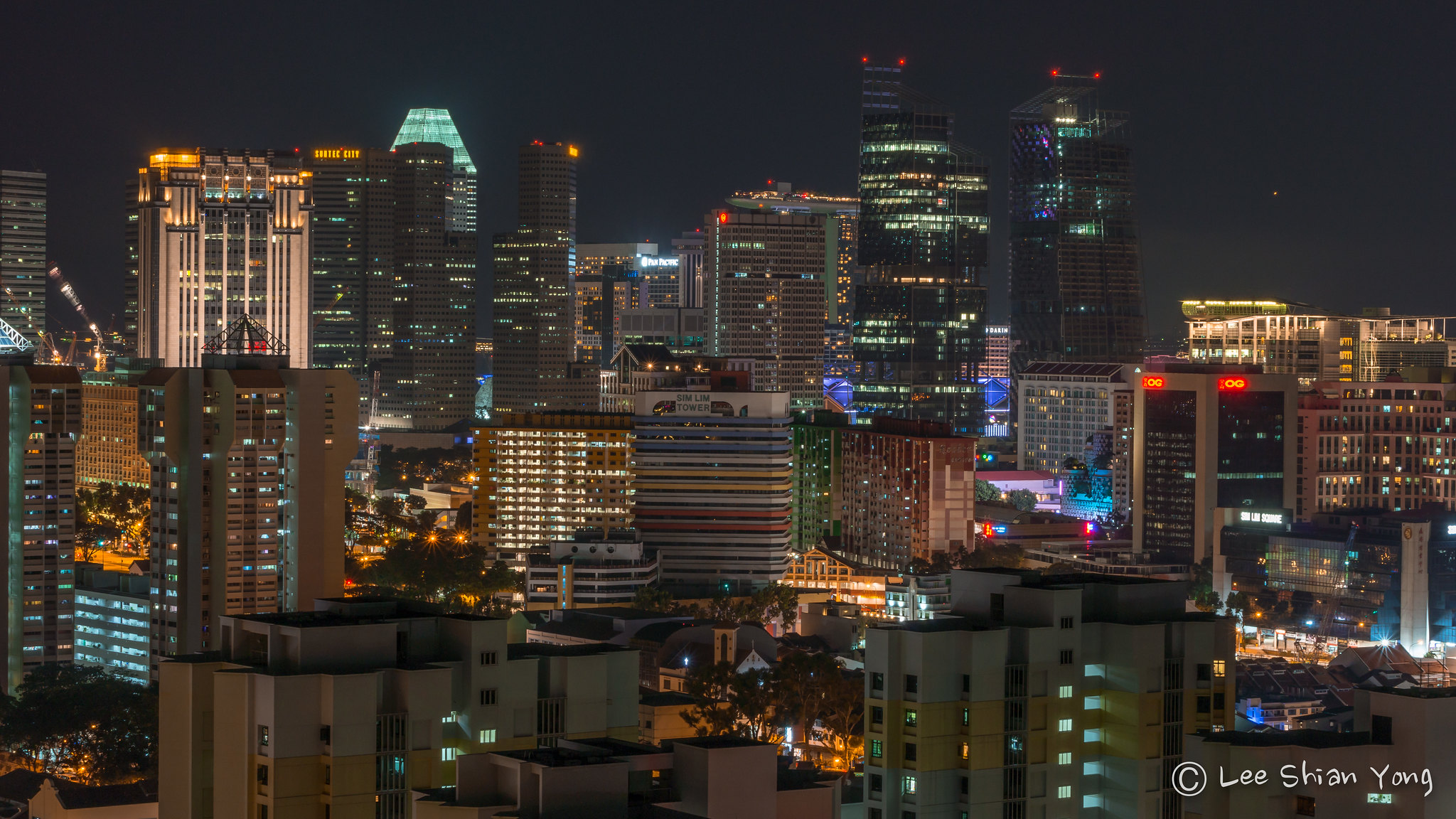This photograph, framed in a horizontal rectangular shape, captures a vibrant city skyline at night, viewed from an outdoor vantage. The top one-third of the image features a dark navy blue sky, its hue softened by the ambient light spilling from the myriad of illuminated buildings below. The skyline consists of both towering skyscrapers and shorter structures, each uniquely adorned with a mix of blue, orange, white, and red lights. Some buildings have their exteriors lit, while others glow from the light within their windows. Neon signs punctuate the scene, and a prominent building on the left side is notable for its exterior screen. In the bottom right corner, the photograph is attributed to Lee Shan Yang, marked by a copyright symbol (©) followed by his name. A subtle red dot in the far right of the sky suggests the presence of an aircraft, further enlivening the night scene.